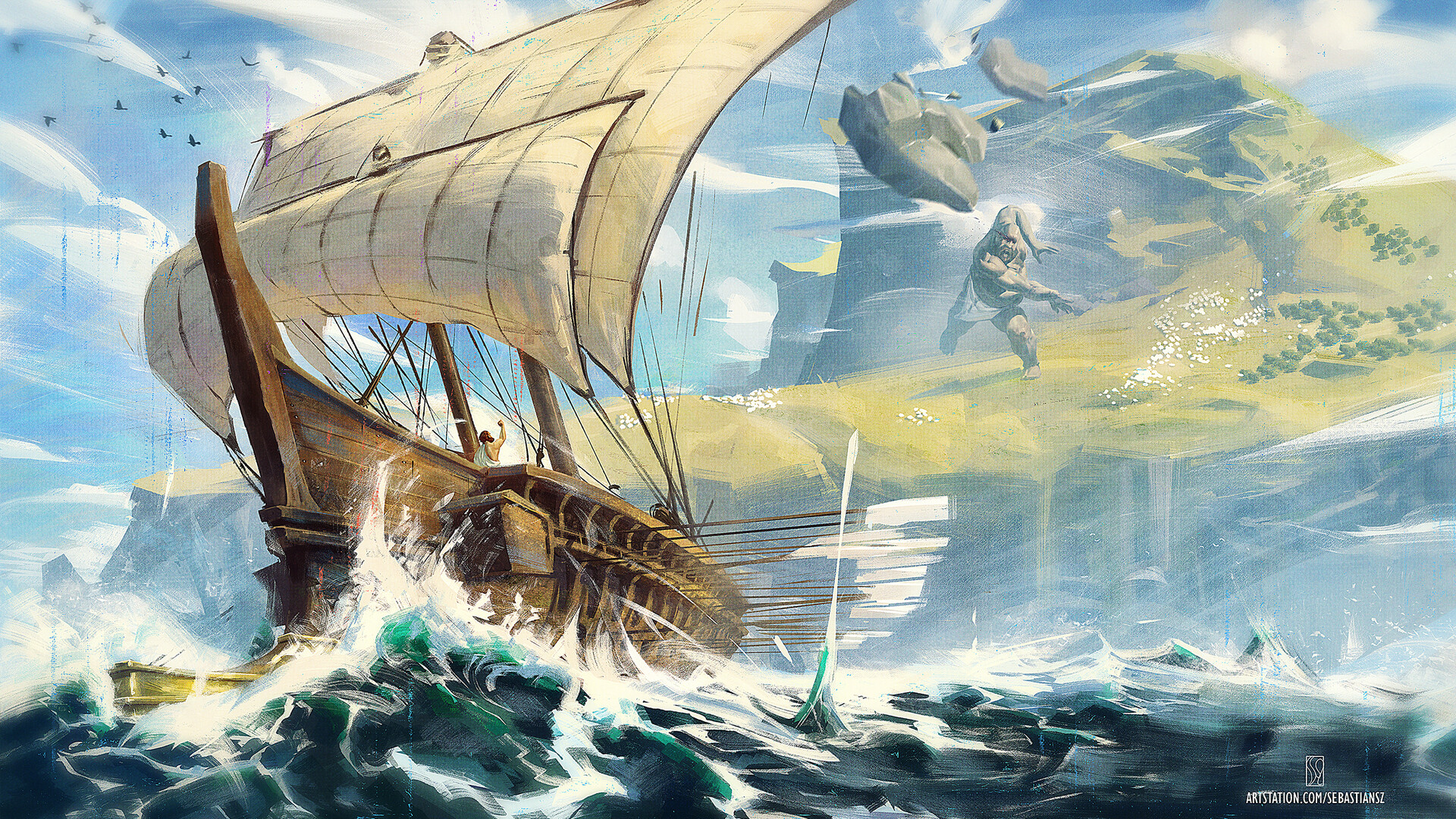This is a detailed fantasy painting in landscape orientation, credited with a watermark "artstation.com/SebastianSZ" and a signature icon in the bottom right corner. The scene depicts a dramatic, stormy ocean with a boat being violently tossed by the rough sea, its white foam splashing into the air. The wind is evident as the sails are billowing, and the numerous oars are splayed outward. A man in a white toga stands on the deck, shielding his face from an incoming massive boulder. In the background, a colossal, grey-skinned giant with a matching beard, clad in a white loincloth with a cross on it, is hurling the boulder from a cliff. The giant is immensely muscular and stands on an outcrop surrounded by trees that appear minuscule next to him. Behind the giant, towering mountains loom, topped with green and dotted with tiny white shapes that might be sheep. The backdrop is a blue sky with visible paint strokes, adding to the dramatic effect of the scene. The boat appears to be fleeing from the barren, grassy island towards the treacherous waters and away from the formidable giant.